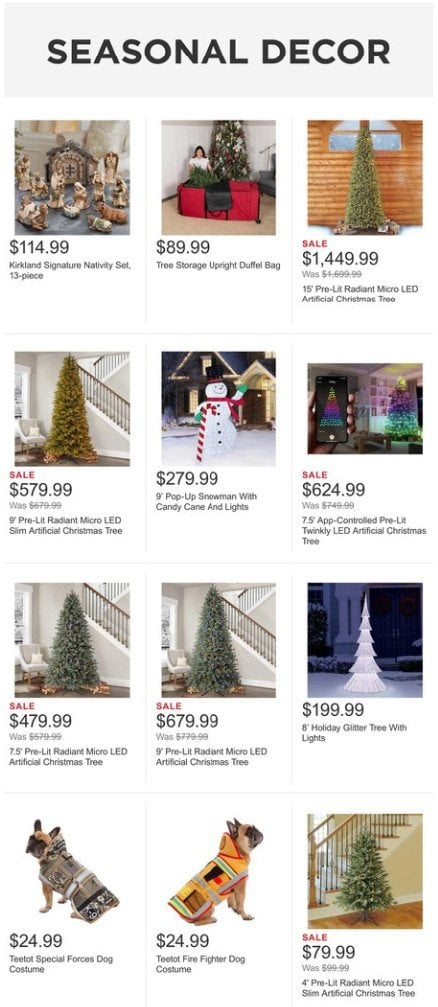The image is a screenshot of a website displaying a selection of seasonal decor items predominantly for Christmas. The page features 12 items in total, each presented with their prices, descriptions, and some offering sale prices. 

The items are organized into four rows, as follows:

**Top Row:** 
1. **Kirkland Signature Nativity Set** - A 13-piece nativity set priced at $114.99.
2. **Tree Storage Upright Duffel Bag** - Priced at $89.99, with an image showing a woman placing a Christmas tree into the duffel bag with another tree behind her.
3. **15-foot Pre-Lit Radiant Micro-LED Artificial Christmas Tree** - On sale for $1,449.99 (originally $1,699.99).

**Second Row:**
1. **9-foot Pre-Lit Radiant Micro-LED Slim Artificial Christmas Tree** - Sale priced at $579.99, down from $670.99.
2. **9-foot Pop-Up Snowman with Candy Cane and Lights** - Depicted standing in front of a house and priced at $279.99.
3. **7.5-foot App-Controlled Pre-Lit Twinkly LED Artificial Christmas Tree** - On sale for $624.99, previously $749.99.

**Third Row:**
1. **7.5-foot Pre-Lit Radiant Micro-LED Artificial Christmas Tree** - Sale priced at $479.99, originally $579.99.
2. **9-foot Pre-Lit Radiant Micro-LED Artificial Christmas Tree** - Sale priced at $679.99, originally $779.99.
3. **8-foot Holiday Glitter Tree with Lights (all white)** - Priced at $199.99.

**Bottom Row:**
1. **Tea-Tot Special Forces Dog Costume** - A khaki and camo dog costume priced at $24.99.
2. **Tea-Tot Firefighter Dog Costume** - Another dog costume priced at $24.99.
3. **4-foot Pre-Lit Radiant Micro-LED Slim Artificial Christmas Tree** - On sale for $79.99, previously $99.99.

The majority of the items are Christmas-themed, with the exception of the two dog costumes. The screenshot does not reveal the website's interface, browser, or operating system details but focuses solely on showcasing the listed products.